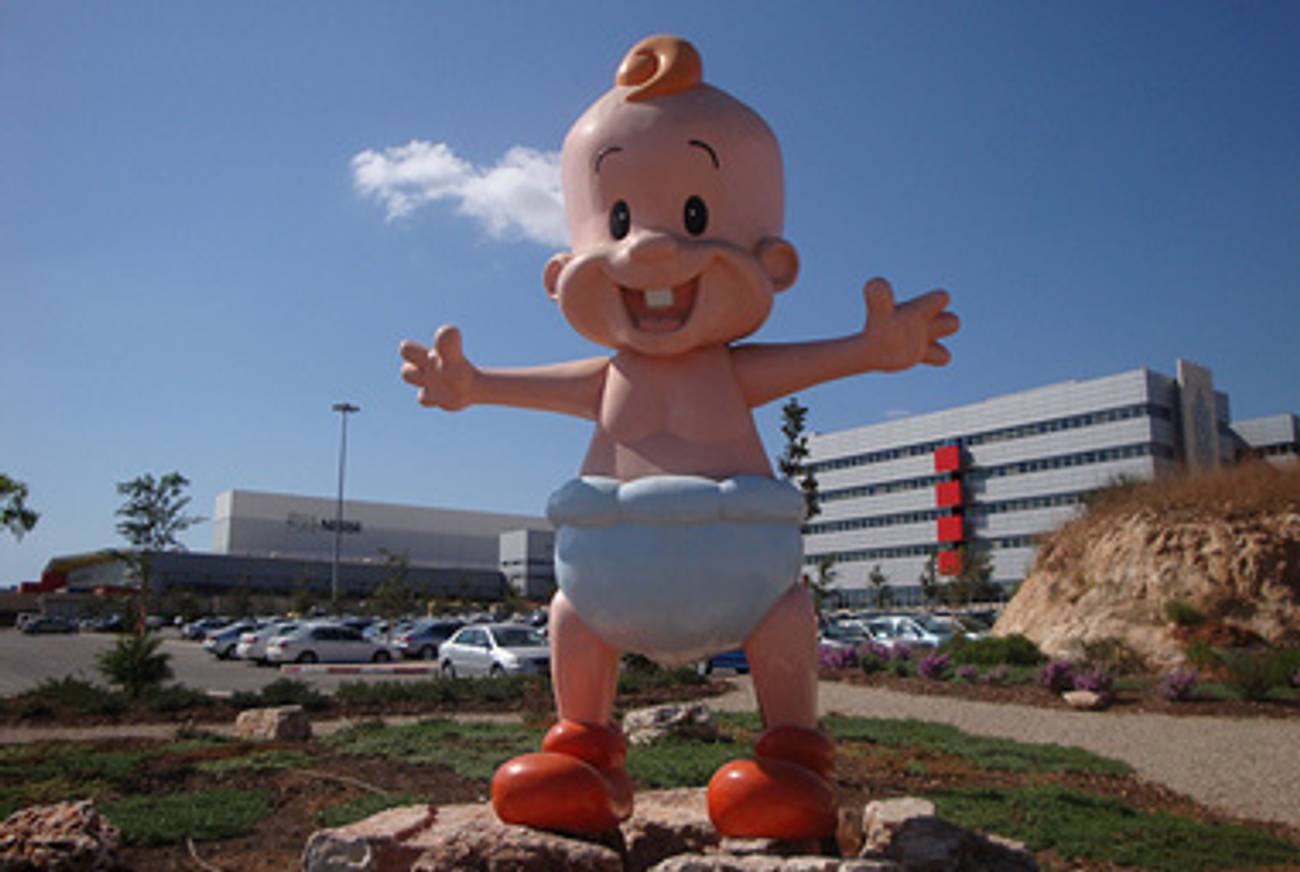The photograph, taken outdoors, showcases a whimsical and oversized statue of a cartoonish baby, likely made of fiberglass. The baby stands on a rocky pedestal amidst a bed of mulch interspersed with greenery. The statue, which seems to be about 10 or 12 feet tall, features a single lock of bright orange hair atop an otherwise bald head, a gleeful expression with an open mouth revealing a single tooth, and wide, black eyes. The baby’s arms are outstretched, as if reaching for a hug, with each hand having a thumb and three fingers. It is dressed only in a large, poofy white diaper and bright red shoes. The figure is positioned slightly angled to the left but predominantly facing the viewer. In the background, a scene typical of a commercial area or car dealership is visible, including a large parking lot filled with cars, various commercial buildings, a small gravel path, and grassy areas. To the right, there is a hillside adorned with purple bushes and a significant building with four red squares. The overall composition captures the exuberant and playful nature of the statue against a bustling backdrop.